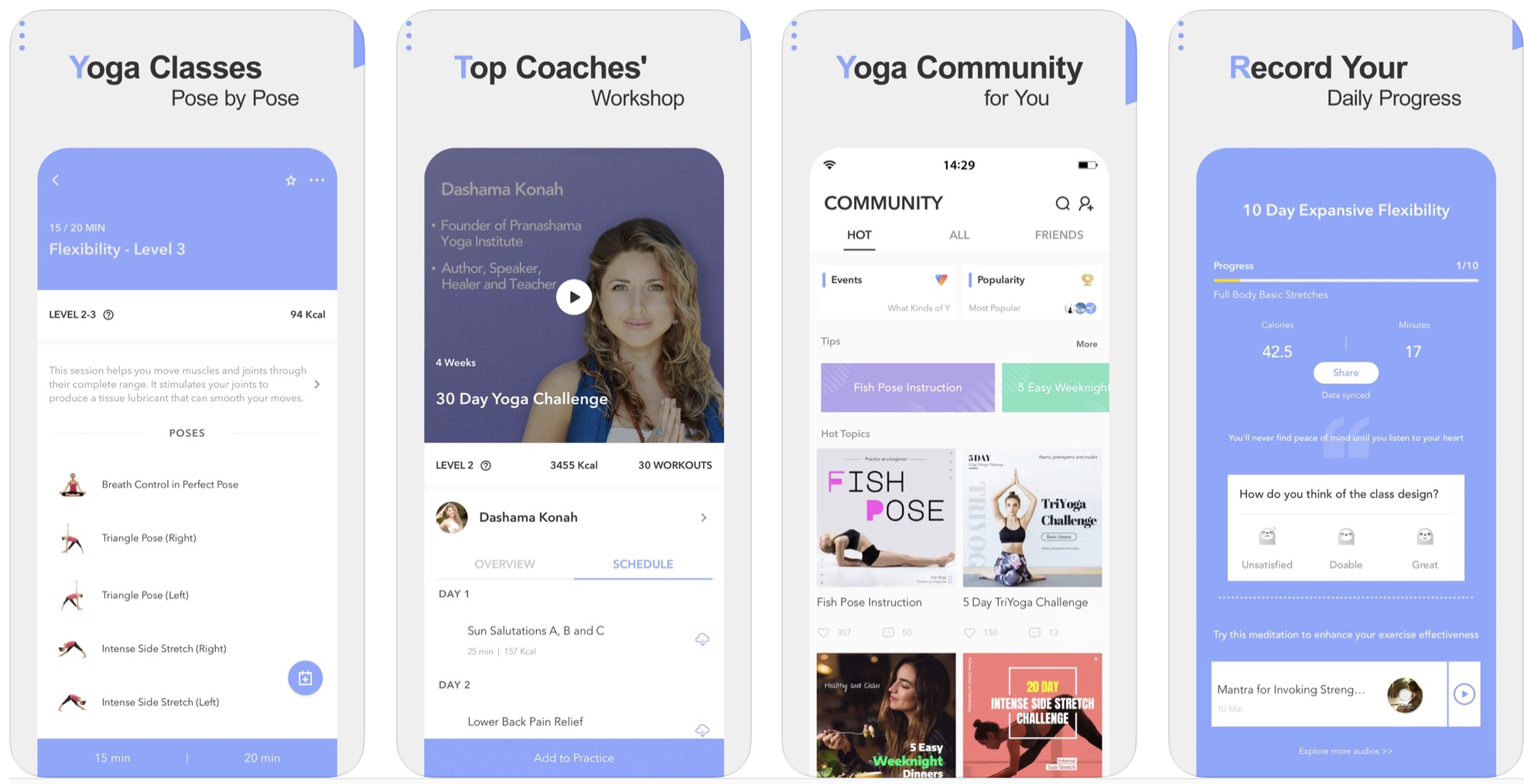Here are concept pages for a yoga app displayed side-by-side, following a left-to-right arrangement. Each page mimics the appearance of a smartphone, featuring a gray background highlighted with bluish-purple accents. These accents include three dots in the upper left corner, a small angular section in the upper right, and various elements such as buttons and backgrounds within the pages.

Each page bears a title at the top, highlighted in bluish-purple, with the remainder of the text in black. The four titles from left to right are "Yoga Classes," "Pose by Pose," "Top Coaches Workshop," and "Yoga Community for You."

**Page 1: Yoga Classes**
- The section begins with the headline "Flexibility Level 3."
- Above the headline, there's information indicating a duration of 15/20 minutes, set against the bluish-purple background.
- Below this is a white background listing a series of yoga poses. Each pose is represented with a small image on the left and its name on the right.
- The difficulty level is indicated as "Level 2 to 3," burning 94 kcal.
- At the bottom, there are buttons for 15 and 20 minutes displayed in light purple.

**Page 2: Pose by Pose**
- A headshot video features the instructor Dashama Kona, founder of the Pachen Ma Yoga Institute, who is also an author, speaker, healer, and teacher.
- Below the video, the start of a weekly schedule is outlined, showing Day 1 and Day 2 for this instructor.
- The schedule menu is selected and highlighted in bluish-purple.

**Page 3: Top Coaches Workshop**
- The headline "Community" is followed by a grid layout resembling album covers, with four items visible.
- Titles include "Fish Pose Instruction," and "5-Day Try Yoga Challenge." The remaining two are obscured but depict images: one of a person eating in a dark restaurant and another of a person performing a yoga pose against a pink background.

**Page 4: Record Your Daily Progress**
- This page displays a progress recording interface predominantly in light bluish-purple.
- The text "10-Day Expansive Flexibility" is featured, along with a progress bar approximately 10% full, with the filled portion highlighted in yellow.
- Options for feedback on the day's class include "Unsatisfied," "Doable," or "Great," along with additional informational elements.

Each page combines functionality with aesthetic design, providing users with a comprehensive and visually engaging interface for their yoga journey.